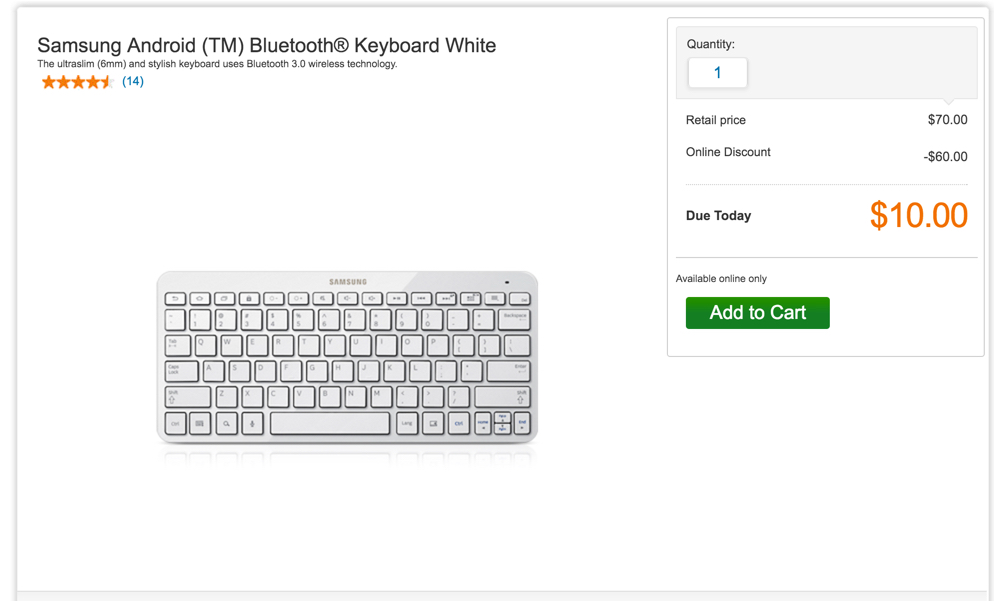The image depicts a web page reminiscent of Micro Center's design, known for its familiar buttons and layout, though it lacks specific branding. The web page features a product description for a white Samsung Android Bluetooth keyboard. This ultra-slim, 6mm thick, stylish keyboard uses Bluetooth 3.0 wireless technology and boasts a rating of 4.5 stars based on 14 reviews, which can be accessed by clicking the number 14. 

On the right side of the page, there is a box displaying purchase details: the input quantity is set to 1, the retail price is $70, and an online discount of $60 is applied, making the total due today $10. The $10 figure is highlighted in orange for visibility. Additionally, there is an "Add to Cart" button. The product is noted to be available online only.

Centrally located in the image is the keyboard, which lacks the numpad and navigation keys, but retains the function keys. It has a minimalist, flat design, consistent with its described slimness. The keyboard is entirely white, showcasing the Samsung logo at the top, aligning with the product details described on the web page.